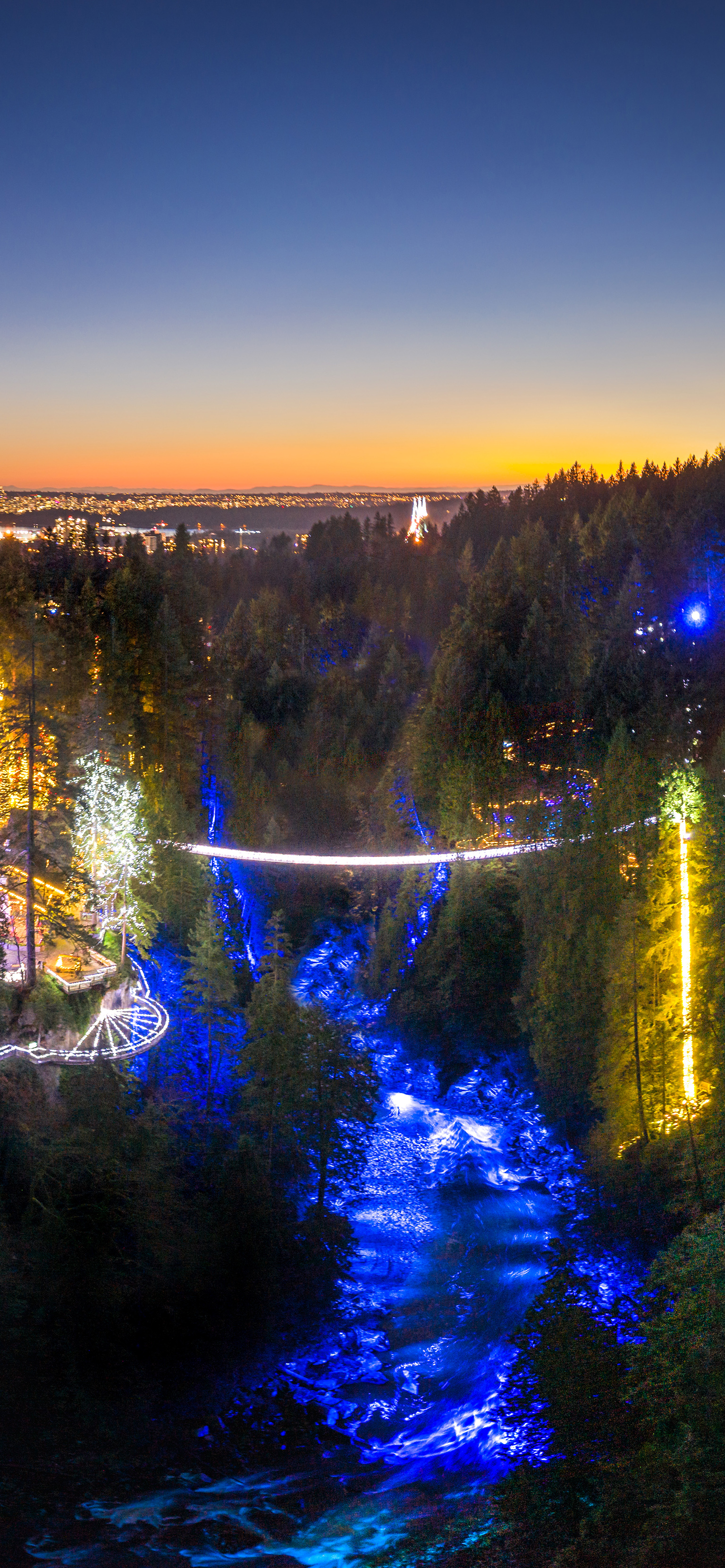The image captures a tall, vertically-oriented, rectangular frame showcasing a vibrantly illuminated landscape scene, likely during twilight or night. It prominently features a striking blue pathway resembling a waterway running through the middle of the scene, bordered by densely packed green pine trees on both sides. On the right side, a glowing yellow light emanates from the ground and travels up one of the trees, contributing to the festive ambiance of the scene. A white-glowing bridge spans the waterway in the center, adding to the intricate light decorations. In the distance, a bright expanse on the left side reveals faint outlines of a city marked by numerous small, distant lights. Above, the sky reflects the soft hues of either a setting or rising sun, enhancing the landscape’s enchanting atmosphere.